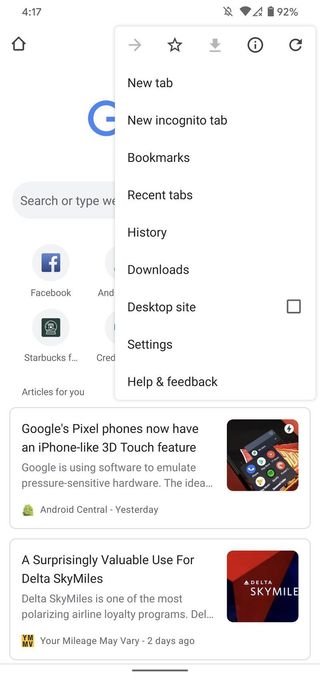This is a screenshot of a Google home page taken on a cell phone. The time displayed on the phone is 4:17. In the status bar, you can see icons indicating no notifications, active Wi-Fi connection, cell phone reception, and a battery level at 92%. 

A Google tab menu has been opened, revealing options such as 'New Tab', 'New Incognito Tab', 'Bookmarks', 'Recent Tabs', 'History', 'Downloads', 'Desktop Site', 'Settings', and 'Help and Feedback'. 

Due to this pop-up menu, only a part of the Google logo is visible, along with the upper portion of the search bar. Below the search bar, icons for Facebook and Starbucks are noticeable. In the "Articles for You" section, there is an article mentioning the new feature in Google's Pixel phones that mimics the 3D Touch feature found in iPhones.